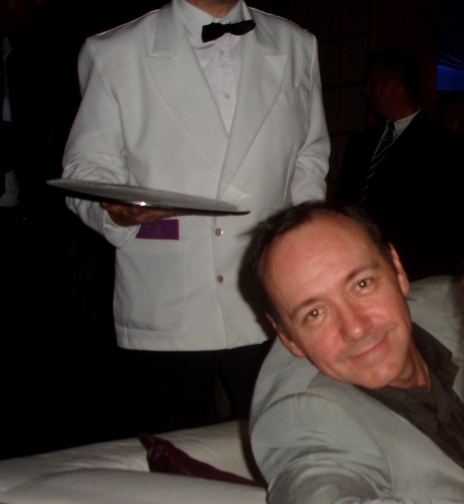In this candid image, actor Kevin Spacey is prominently positioned in the center, sitting on a white sofa with a blue or purple pillow. He is dressed in a gray suit paired with a black shirt, and he displays a sarcastic smile as he looks directly into the camera, his brown eyes reflecting the flash. Beside him, a waiter dressed in a white tuxedo with an oversized jacket, white button-down shirt, and black bow tie holds a silver tray. The background is very dark, suggesting the setting might be a dimly lit room or an outdoor night event, with various people in suits moving about in the background. The scene has an air of a gathering or a party, enriched by the contrasting colors of black, white, gray, tan, silver, and maroon visible in the image.